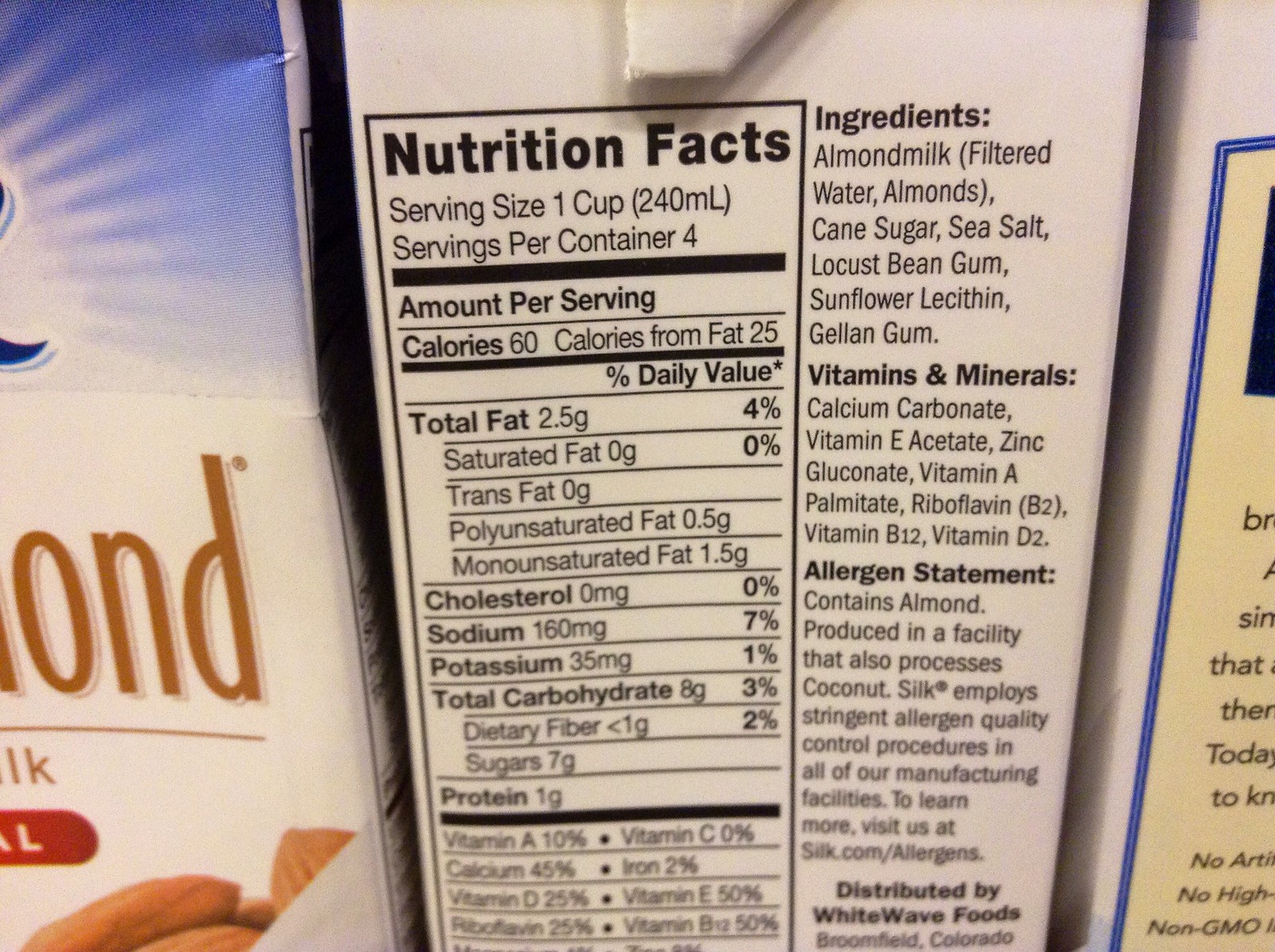This photograph showcases the back panels of three cardboard cartons, primarily focusing on one in the center, which is a carton of almond milk. The center carton is rectangular and displayed in a portrait orientation with a white background featuring black lettering. The nutritional facts, ingredients, vitamin and mineral content, and allergen statements are clearly listed. Key ingredients include almond milk, filtered water, almonds, cane sugar, sea salt, locust bean gum, sunflower lecithin, and gellan gum, alongside various vitamins and minerals. The bottom of the carton displays a "Distributed by WhiteWave Foods" note.

To the left, another carton, also identified as almond milk, displays "OND" and is decorated with large almond visuals at the bottom, a white base, brown lettering, and blue rays at the top. The third carton on the right, partially visible, has a yellow background framed in white with a blue border and features some black lettering that is not entirely readable.

Overall, the image effectively highlights the nutrition panel in the center and two adjacent cartons, providing various perspectives and detailed labeling information of the almond milk products.